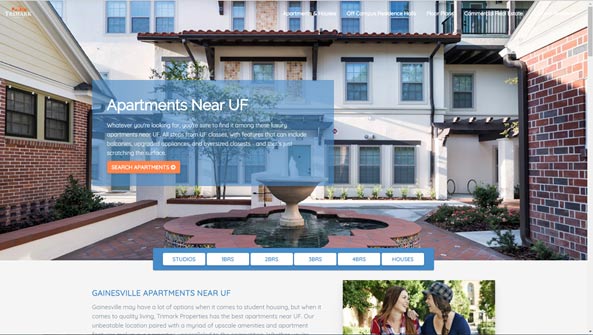This image showcases a stately three-story or possibly taller white building in the background, complete with a couple of shade structures. Flanking the central area, where a fountain gracefully stands, are two single-story brick structures. Overlaying the image, in a transparent blue box, is white text that reads, "Apartments near UF. Whatever you're looking for, we're sure to find it." Accompanying this call to action is an orange button labeled "Search Apartments." At the bottom of the image, a navigation bar lists various living options: studios, one bedrooms, two bedrooms, three bedrooms, four bedrooms, IDRAs, and houses. Below the navigation bar, the text "Gainesville Apartments near UF" is displayed next to a picture of two women sharing a laugh, looking at each other warmly.